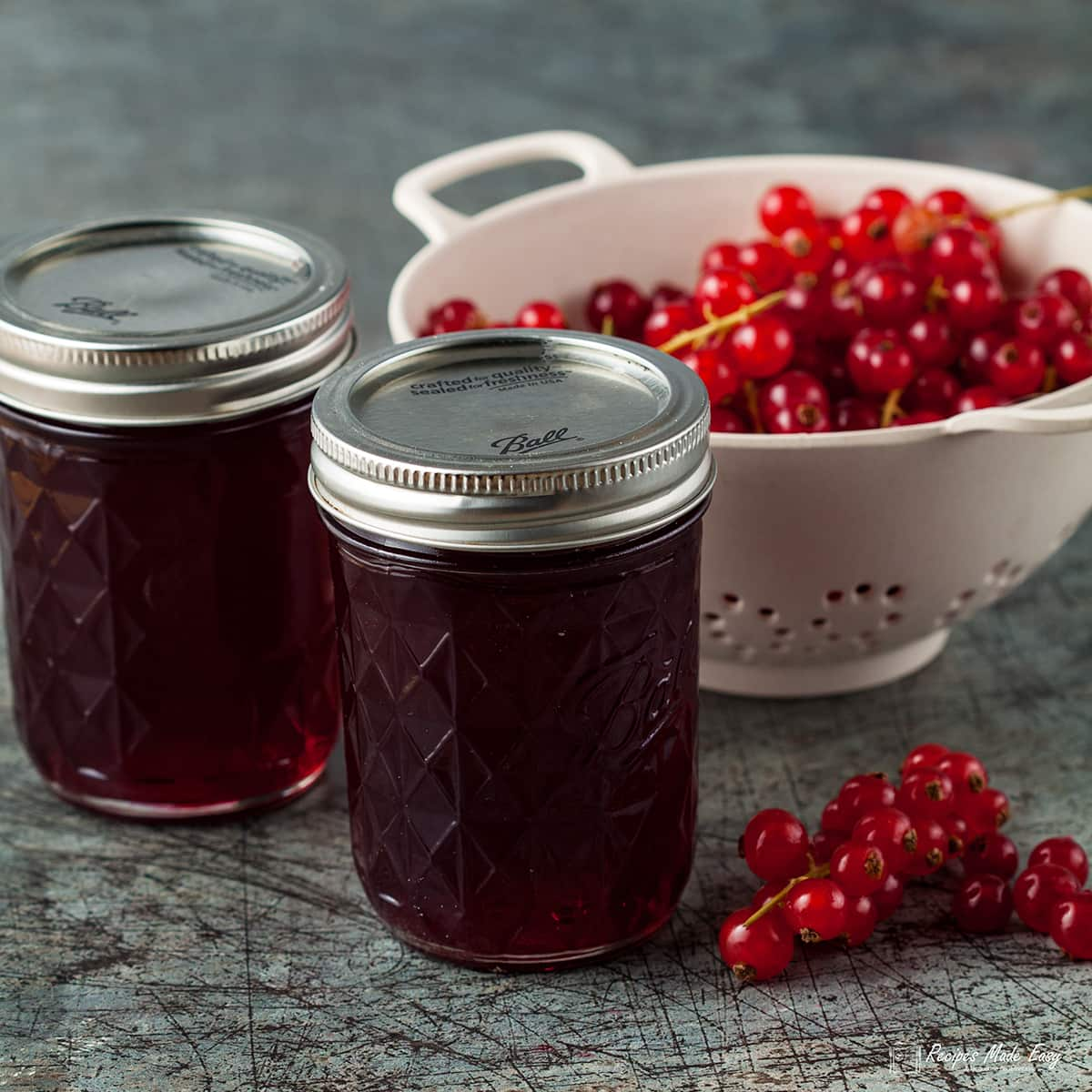The image features a white colander bowl, designed with holes midway up its sides for rinsing produce, and is filled with vibrant cherry red berries identified as red currants. Each currant is attached to a small twig-like vine and has a tiny black stem at its end. The colander is set on a rustic blueish-gray table that bears signs of wear, such as scattered marks and scrapes. Beside the colander, there are two pint-sized mason jars containing a dark red jam or jelly, sealed with metal lids and rings, indicating they have been properly canned. To the bottom right of one jar lies a small bunch of red currants, adding to the scene's detailed and homely charm.